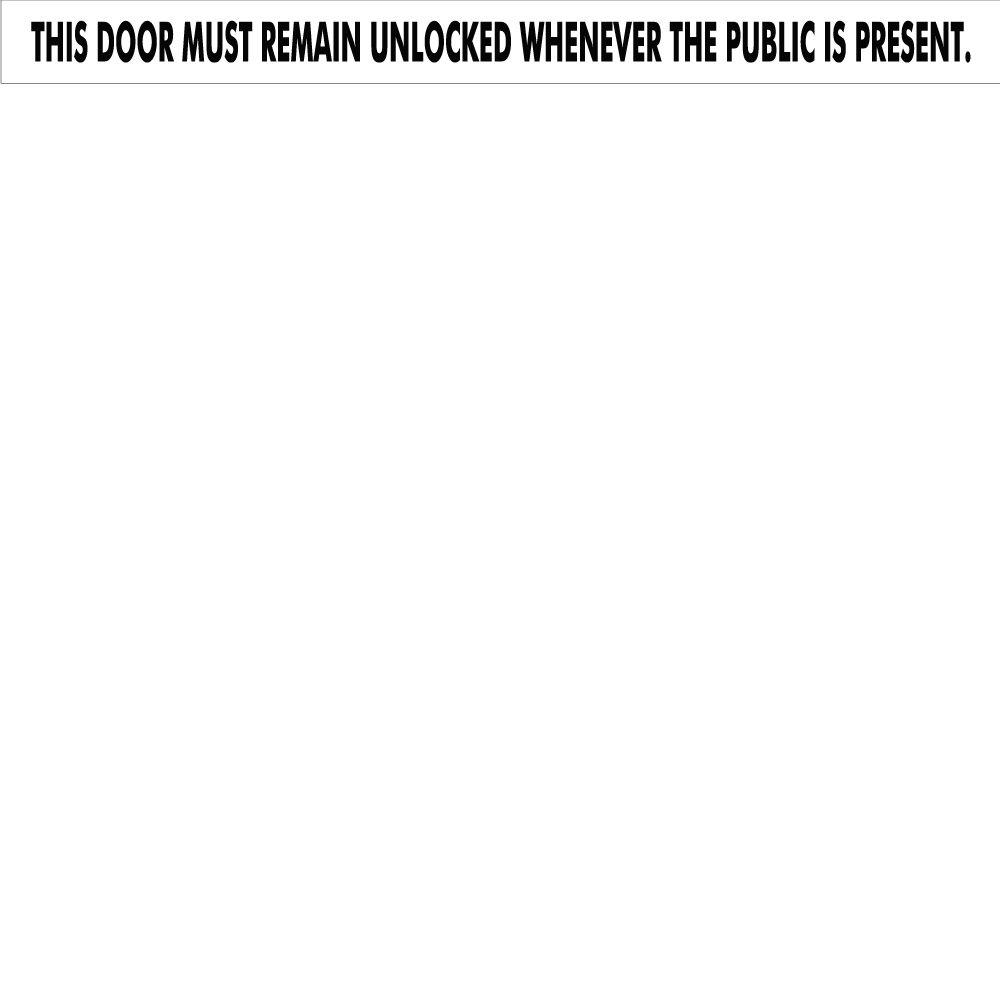The image features a rectangular sign with a gray border and a white background. At the center of the sign, there is a bold and capitalized message in black text that reads: "THIS DOOR MUST REMAIN UNLOCKED WHENEVER THE PUBLIC IS PRESENT." The words are spaced out distinctly, giving the text a stretched appearance. The sign's purpose is clearly conveyed, ensuring that it catches the attention of anyone nearby.